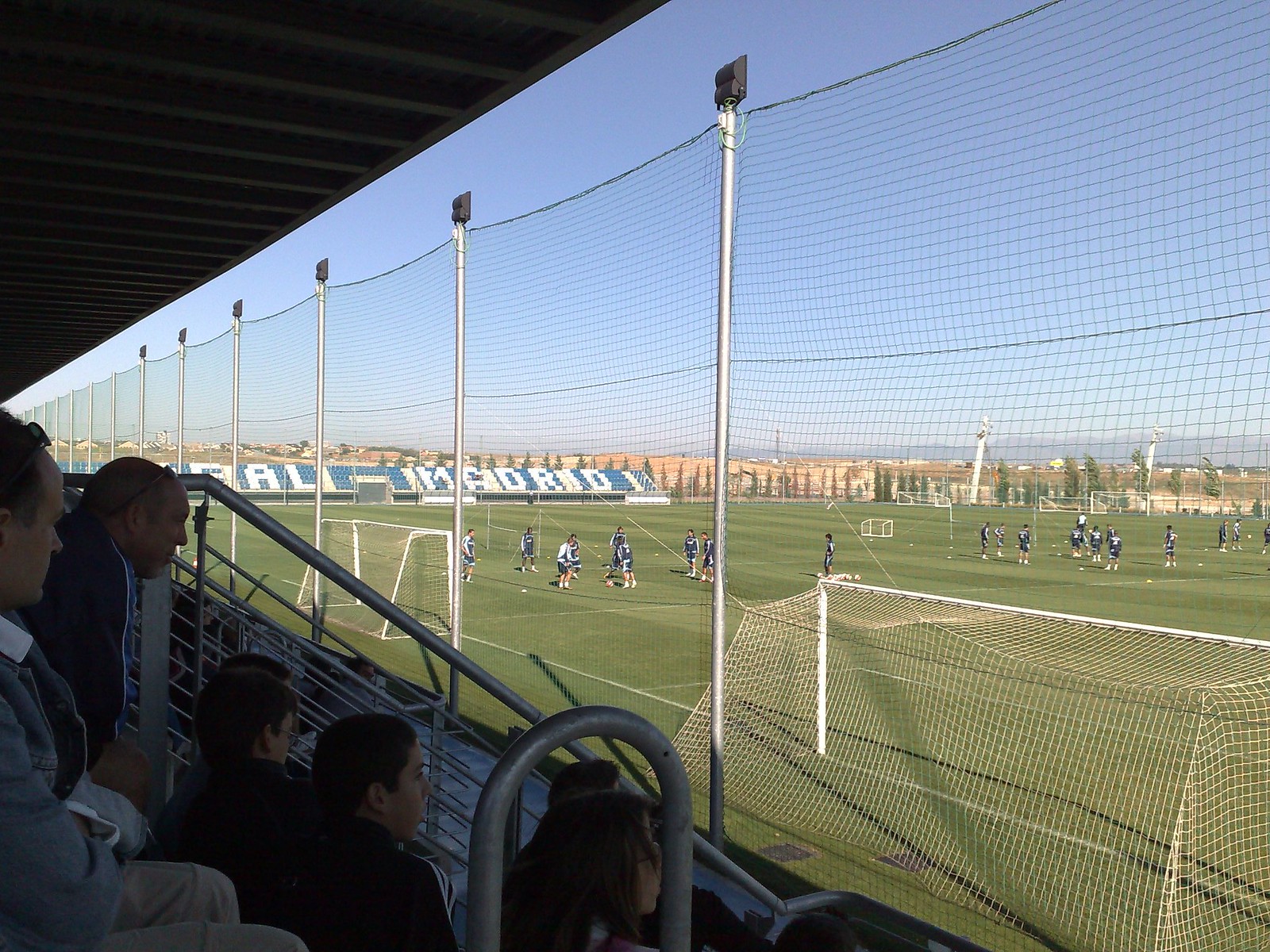The image captures a bright and sunny day at a large, outdoor soccer field set against the backdrop of a distant mountain range and hundreds of trees. The photo is taken from the spectator stands, which are covered by a roof and feature metal railings. A handful of spectators, possibly parents, sit in chairs, watching the scene unfold. A substantial 20-foot net stretches across the front of the spectator area, attached to poles and studded with lights, presumably to protect viewers from stray soccer balls.

On the field below, multiple soccer goals are set up, indicating several adjacent fields, likely for tournament-style play. Numerous soccer players, dressed in various shades of blue and white uniforms and jackets, are scattered across the green expanse, seemingly engaged in practice or warm-up drills, as the field is dotted with soccer balls. The image suggests an organized yet relaxed atmosphere, preparing for more formal play, all under a mostly blue sky.